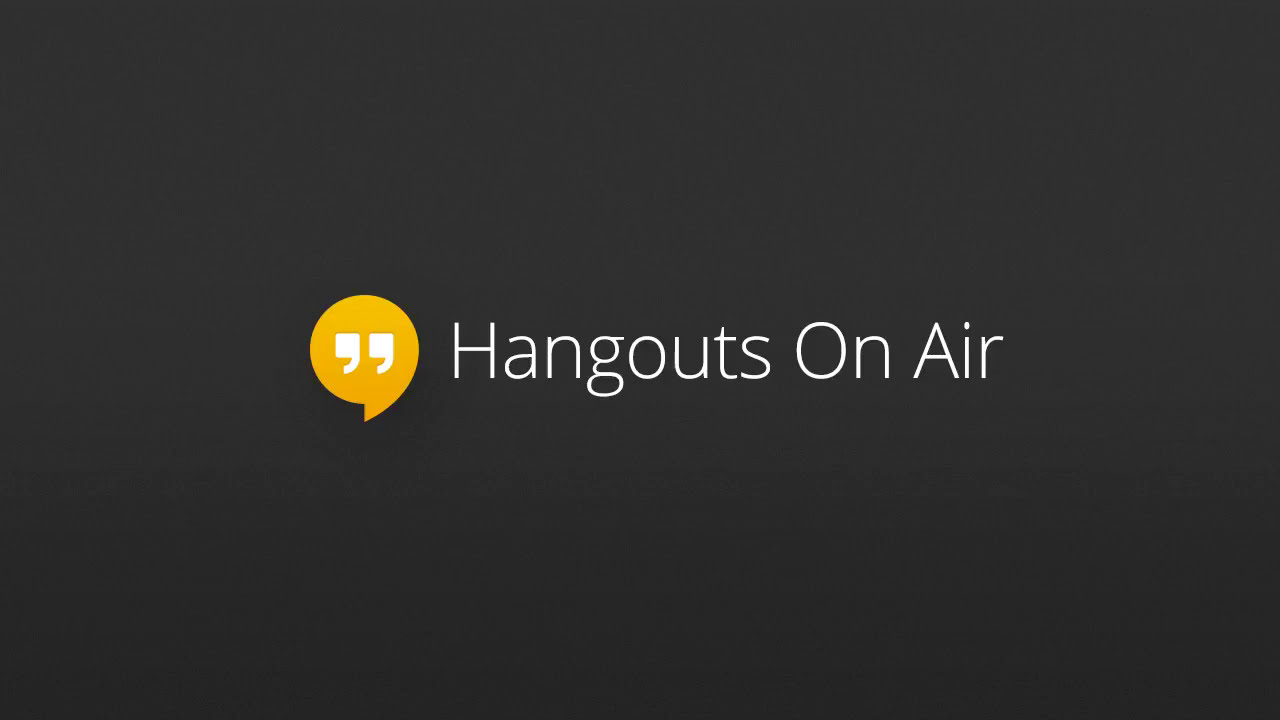The image features a centrally placed, clean white text that reads "Hangouts on Air" in regular, non-bold font. To the left of this text is a yellow speech bubble containing white quotation marks. The entire background is a solid gray. This simplistic design, possibly a screenshot for a video header or a website element, emphasizes the logo of "Hangouts on Air" with its capitalized H, O, and A, against the contrasting backdrop.